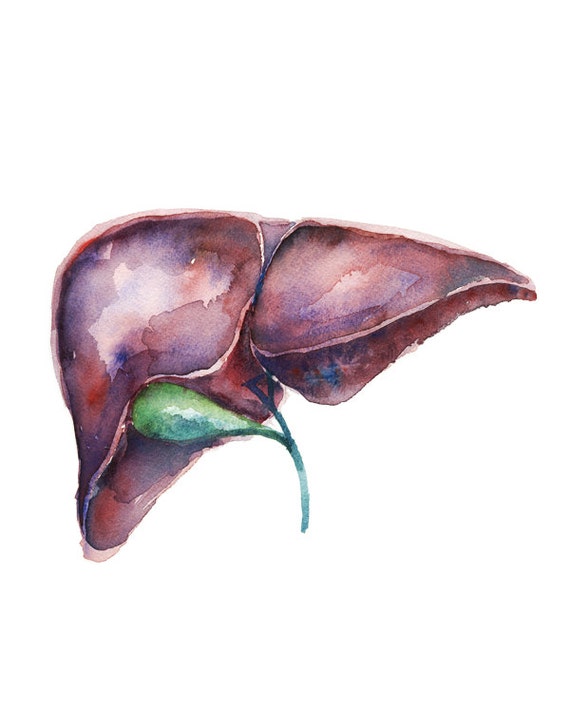The image depicts a watercolor painting set against a clean white background with no text or borders. The painting features a strikingly slender green stem that extends upward and ends in a large, bulbous green bud. The bud supports two massive, oddly shaped petals. The petals, which are colored in a medley of red, white, blue, pink, purple, and off-white, are oversized to the extent that they almost resemble helmets. These petals are attached at various angles, giving the artwork a somewhat triangular shape that spans the upper left corner and the left side of the painting. Despite its abstract appearance, the painting retains some identifiable features of a flower. The stem, thin and green with hints of white and blue, adds to the abstract, yet recognizable, floral composition. The artist’s intention seems to lean towards a non-realistic representation, emphasizing watercolor’s intrinsic fluidity and ethereal quality.